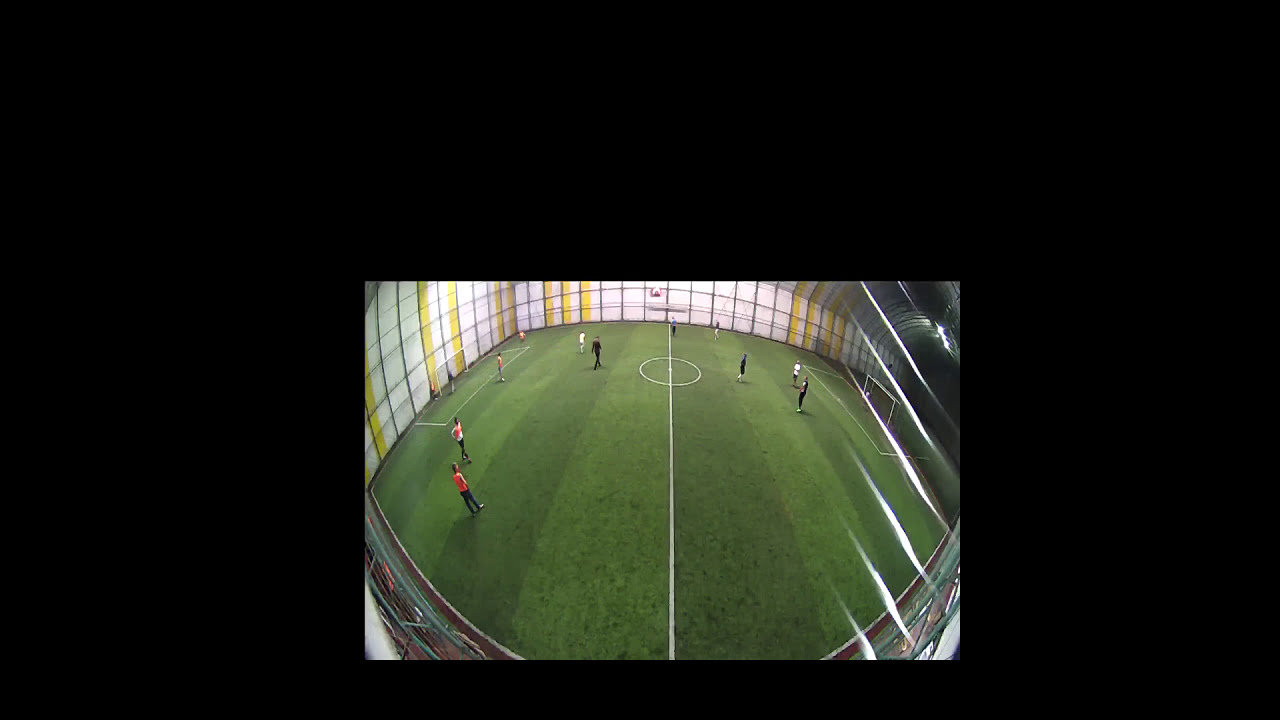The image features a fisheye-lens photograph of an indoor soccer field with dark and light green stripes. A prominent white line runs through the center of the rectangular field, with a white circle marking the midfield. The picture is taken from an elevated angle, offering an above view of the field. There are eight to ten players visible: some wearing orange shirts, others in white or black uniforms. Four players in orange are located on the left side, a white and a black-uniformed player are on the right half, and three black-uniformed players along with another white-uniformed player are near the goal. The indoor setting includes walls with yellow stripes over a white background and some lights are mounted on the walls. The field is enclosed, with no spectators visible. The time appears to be nighttime, inferred from the darkness seen in the top right of the image. The image is bordered by a thick black frame on the top, left, and right sides, while the bottom border is considerably narrower. The overall color palette includes black, white, yellow, gray, green, red, maroon, and tan.